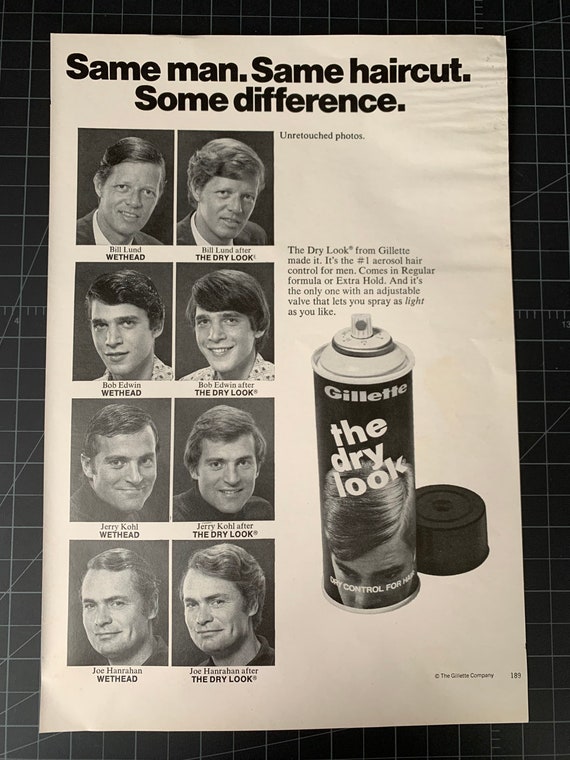This black-and-white advertisement, likely from the 1970s and positioned on a graph paper-style background, promotes "Gillette: The Dry Look," a dry control spray for hair. The top of the ad features the bold text, "Same man, same haircut, some difference," illustrating the contrasting hairstyles—wet head versus dry look—on four different individuals. Each man is shown twice, once with wet hair labeled "wet head" and again with hair styled using "the dry look" from Gillette, resulting in fluffier, well-groomed appearances. The individuals vary in age: a teenager, two men in their 30s, and an older man, displaying the product's versatility across age groups. The right side of the ad prominently features an uncapped spray can with a graphic silhouette of a man's head and the text, "Gillette: The Dry Look. Dry control for hair," alongside a description that highlights its status as the number one aerosol hair control for men. The text also notes that the spray comes in regular or extra hold and is the only one with an adjustable valve for customizable application. This advertisement is identified as being from page 189 of an unspecified magazine.